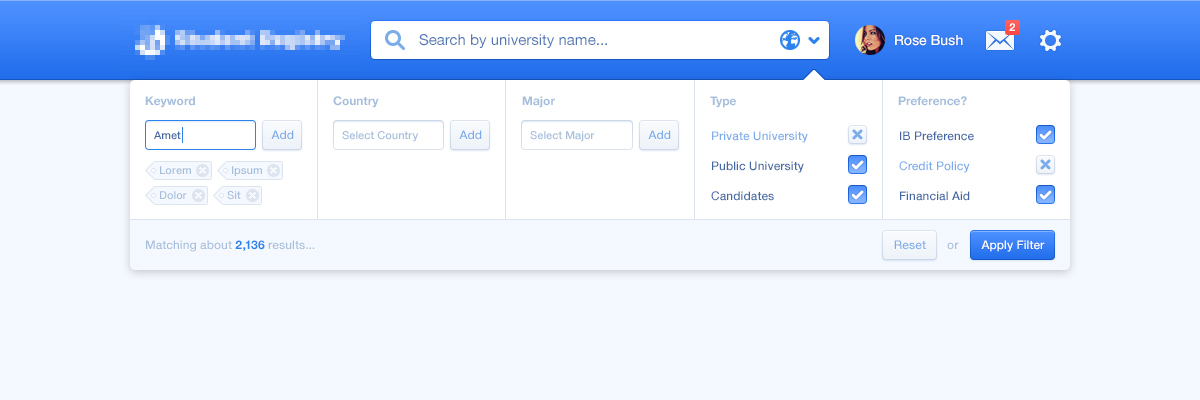A screenshot from a website features a blue rectangular interface that is slightly blurred in the top left corner, obscuring the company name. Dominating the upper section of the image is a white rectangular search box, prompting users to "Search by university name." To the right of this search box, a small circular avatar displays a person's picture with the name "Rose Bush" beside it. Adjacent to the name is a small white envelope icon with a red notification badge indicating the number 2.

Beneath this, there is another white rectangular section divided into five labeled blocks for input and selection. The first block is labeled "Keyword," featuring a search box with "A-M-E-T" pre-entered and an "Add" button next to it. The second block is labeled "Country," containing a dropdown that says "Select country" and an accompanying "Add" button. The third block is labeled "Major," with a similar dropdown stating "Select major" and its respective "Add" button.

The fourth block is labeled "Type," providing options for Private University, Public University, and Candidates, each with its own checkbox. An 'X' marks the box beside Private University, while the checkboxes for Public University and Candidates are filled with blue and white checkmarks, respectively.

The fifth block is labeled "Preference," bearing a question mark icon and options for IB Preference, Credit Policy, and Financial Aid. The IB Preference and Financial Aid options are selected, indicated by blue boxes with white checkmarks. In contrast, the Credit Policy option shows a white box with a blue 'X.'

In the bottom left, the interface indicates that there are "Matching about 2,136 results."